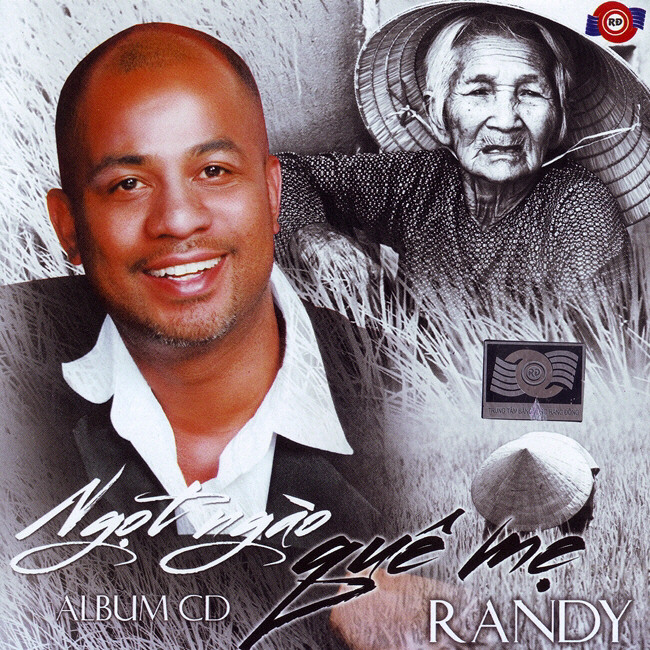The image appears to be a poster or album CD cover featuring a full-color picture of a smiling black gentleman with a bit of facial hair and balding on top. His name, "Randy," is displayed in the lower right-hand corner. The background features a black-and-white photograph of an elderly Asian woman, possibly female, wearing a dark top with dots and a traditional rice paddy hat. She is set amidst a backdrop of tall grass or wheat. An additional image of a similar Asian rice field worker's hat, also in black and white, is located towards the bottom of the cover. The text appears to be in Spanish, but the exact wording is unclear.